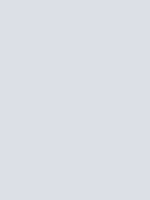Caption: An image displaying a light grayish-purple rectangle with no discernible details or subjects. The entire frame is filled uniformly with the solid color, offering no visible elements to describe or analyze.